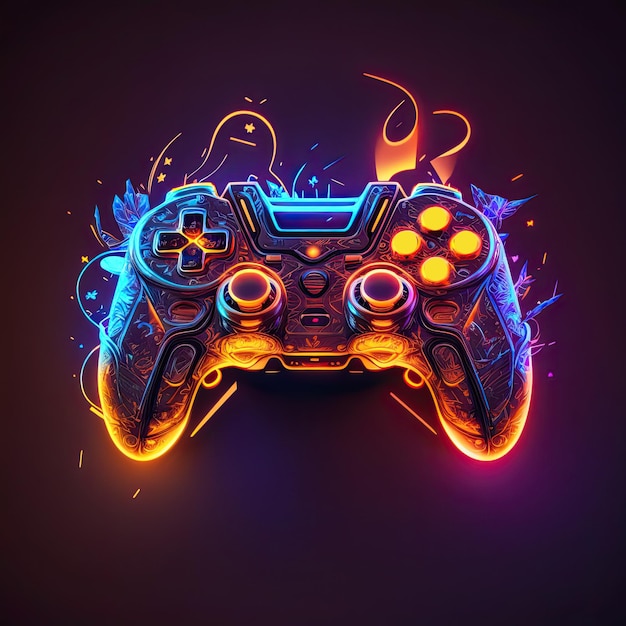This vibrant and intricate poster features an illustrious drawing of a PlayStation controller, prominently set against a very dark, almost black background that accentuates its bright, neon colors. The controller itself, potentially a PlayStation 4 model, exudes a fiery essence with an eye-catching palette of orange, pink, blue, and purple. Flames in maroon and orange hues appear to leap out from behind it, enhancing the impression that the controller is ablaze. Intricate, comic book-like sketches and possible game characters seem to emerge from behind the controller, adding layers of depth and intrigue. Around the controller, small X's or plus symbols create a dynamic pattern in the background. This combination of vivid neon colors and detailed artistry makes the yellow tones particularly striking, while the overall effect suggests a glowing, lively energy, perfect for a teenager who loves video games.